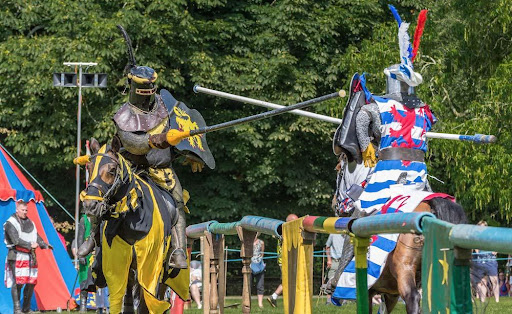This photograph captures the excitement of a lively jousting competition, resembling a renaissance festival. Central to the image are two knights mounted on their horses, charging towards each other on opposite sides of a makeshift fence made from plastic tubing. The knight approaching on the left rides a brown horse and is adorned in an outfit with horizontal blue and white stripes running from his boots to his neck, accented with a vivid red lion standing on its hind legs on his back. His metal helmet is topped with a striking red, white, and blue feather. Clutched in his hand is a long jousting lance with a round tip. The opposing knight, riding a black horse draped in a yellow cover, wears striking black and yellow attire, complete with a black helmet. His shield, also black, bears a yellow animal insignia. Both knights, embodying the essence of medieval chivalry, are equipped with armor and shields as they charge towards one another, lances poised for the clash. A red and blue striped tent marks the background, enhancing the vibrant, historical atmosphere of the event.